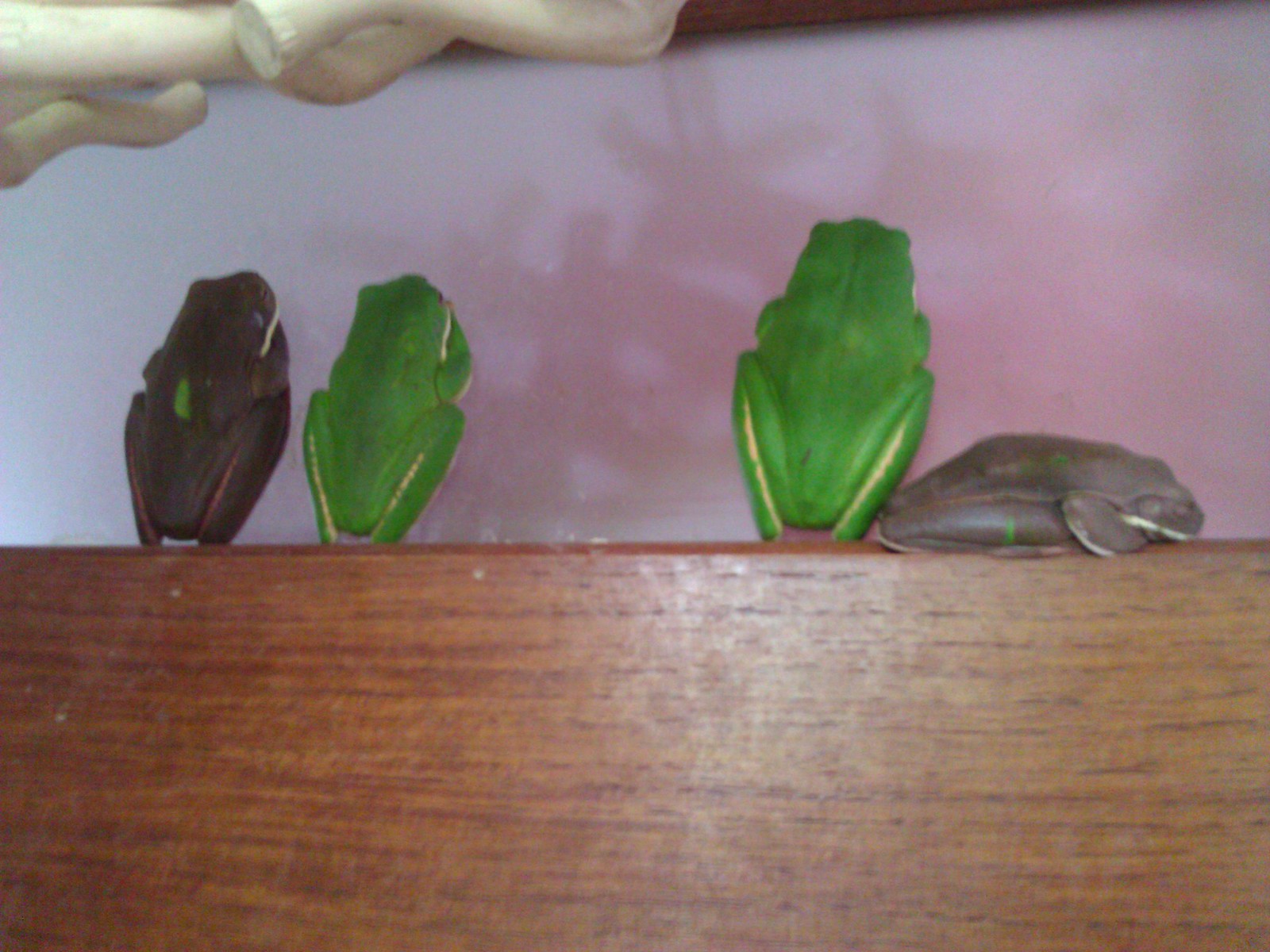The image depicts four small frog sculptures arranged on a polished brown wooden table. From left to right, the first frog is brown, followed by a green frog, and there is a space of approximately two and a half to three inches before a second green frog. The fourth frog on the far right is a subtle gray. All the frogs are facing an opaque background, though the exact nature of the backdrop is unclear. The brown frog on the left is roughly one to one and a half inches in length, while the gray frog on the right is slightly larger, measuring about two inches. A flash of light reflects off the polished table, drawing additional attention to the scene. Additionally, the top of another sculpture can be seen in the upper part of the image, providing an extra element of intrigue to the composition.